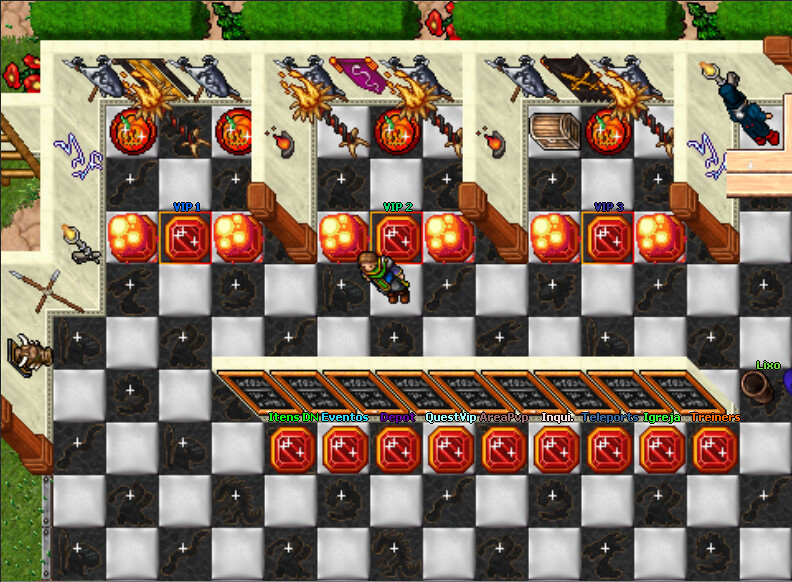The image is a color screenshot from an online, old-school role-playing video game, presenting a nearly bird's-eye view of a game map that features a black and white checkerboard pattern. The scene showcases multiple rooms divided by brown columns and walls, each room adorned with medieval-themed decorations including torches, shields, banners, swords, and coats of armor hanging on the back walls. A player avatar is situated centrally within the layout, giving the sense of active gameplay. Green hedges can be seen at the top of the image, suggesting an outdoor setting bordering the rooms. The overall appearance is reminiscent of classic RPGs like "Zelda," emphasizing a simple yet iconic medieval aesthetic.